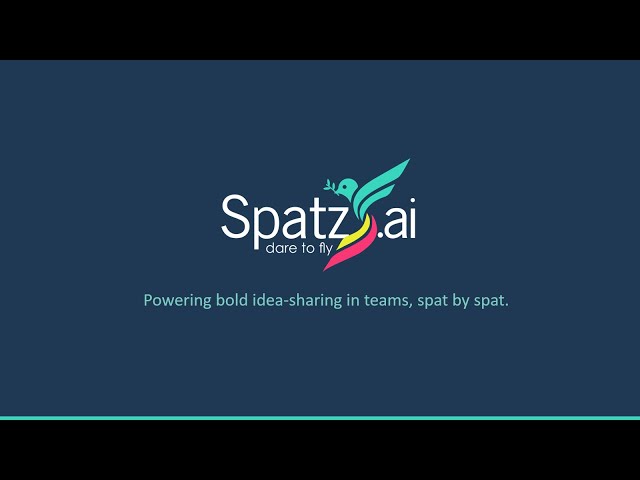This horizontal rectangular image functions as an advertisement for the company SPATZAI. Dominated by dark blue in the center, the image is bordered at the top and bottom by solid black bands. An aqua-colored line separates the dark blue central area from the bottom black band. Prominently featured in large white text at the center is the name "SPATZAI." Between the letters Z and A is an artwork of a flying bird, which boasts teal wings and a head, complemented by a vibrant tail with yellow and red feathers. Below the letters SPATZ, the tagline "Dare to fly" appears in small white text. Further down, another line of text in bluish color explains the company's mission: "Powering bold idea sharing in teams, SPAT by SPAT." The advertisement employs a striking palette that includes dark blue, black, white, teal, yellow, pink, mint green, and gray, creating a visually compelling presentation aimed at promoting innovation within business teams.